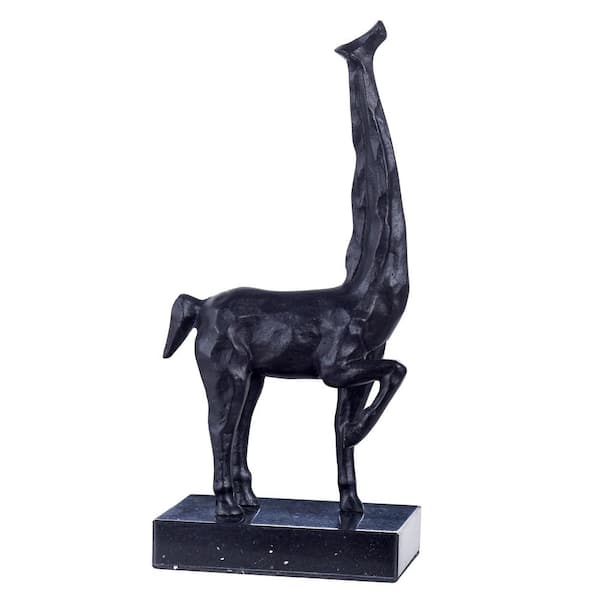This image features a photograph of a striking dark black statue or figurine, prominently set against a completely white background. The artwork, resting on a rectangular black platform about two or three inches thick, depicts a hybrid animal merging characteristics of a horse and a giraffe. The statue showcases four long legs, with three firmly planted on the platform and one bent upwards at the knee in a dynamic pose. The creature exhibits a short tail reminiscent of a horse and an elongated neck akin to that of a giraffe. Notably, the neck concludes with a small stump, indicating the absence of a head, giving the impression of a headless horse. The figure's sleek and shiny surface, potentially crafted from wood or metal, accentuates its muscular form, presenting a robust, well-exercised appearance. Noteworthy is the statue's minimalist detailing, as it lacks sculpted hooves or toes, emphasizing its stylized and abstract artistic nature.